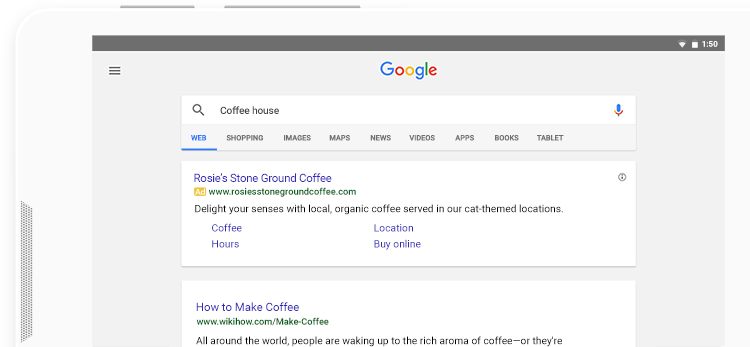The image depicts a Google search results page, and at the very top is a gray navigation bar featuring the Google logo in its characteristic colors of blue, red, yellow, and green. Below the logo is the search bar with the query "coffee houses" inputted. 

Underneath the search bar, there is a horizontal row of category tabs for filtering search results: Web (highlighted in blue), Shopping, Images, Maps, News, Videos, Apps, Books, and Tablets, each tab underlined differently with blue or gray indicators. The Web tab is currently active, highlighted in blue with a blue underline, while the rest of the tabs remain gray.

The search results below show two visible entries, though the second entry is partially cut off. The first result is noted as an ad with the title "Rosie's Stone Ground Coffee," displayed in blue text. Adjacent to the ad label, which is set in an orange box, is the URL "rosiesstonegroundcoffee.com" in green. The ad description reads, "Delight your senses with local organic coffee served in our cat-themed locations." Below the description are links in blue text labeled "coffee hours," "location," and "buy online."

The second visible result has the title "How to Make Coffee" from wikihow.com with the URL "wikihow.com/make-coffee." Its snippet begins with, "All around the world, people are waking up to a rich aroma of coffee or are there..." The snippet cuts off before completing the sentence. Unfortunately, the bottom of the page is also not visible in the image.